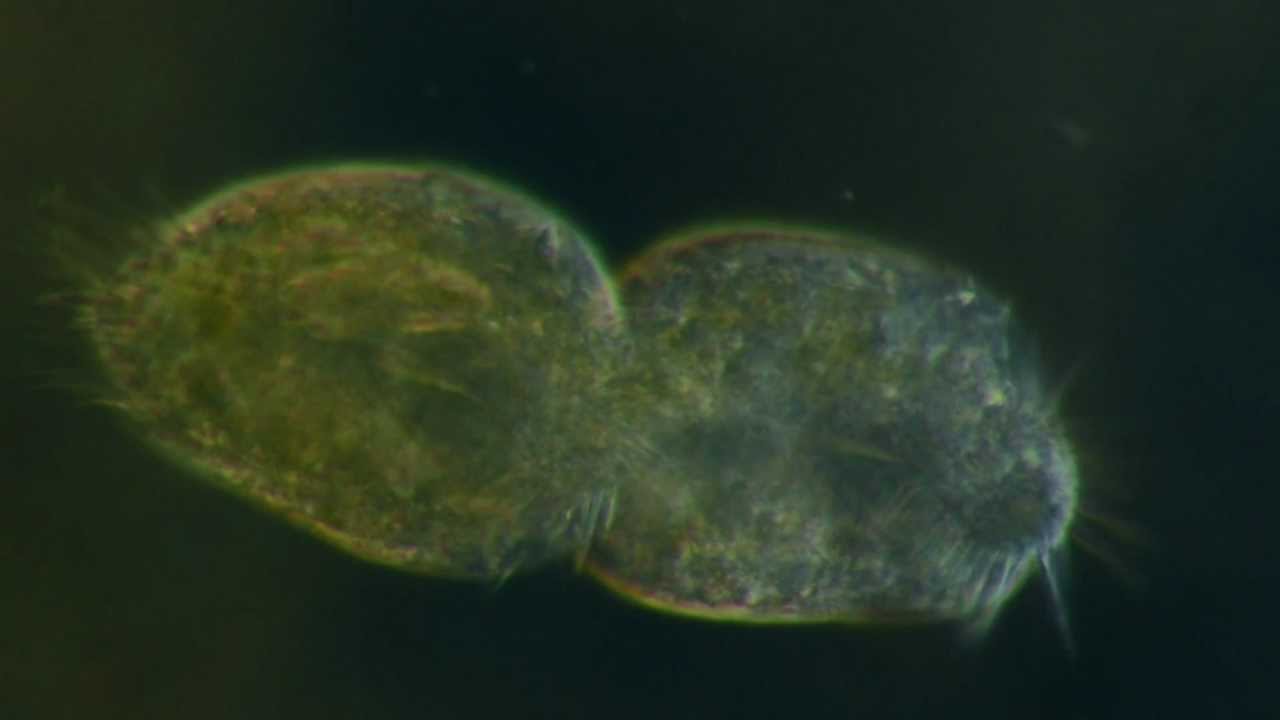This image portrays a highly magnified view of a microscopic life form, possibly a bacterium or amoeba. The organism, somewhat resembling jellyfish, consists of two oval blobs, semi-lumped together. Its dominantly green hue features variations with a slight yellowish tint and darker areas within its body, giving it a fluorescent-like appearance. The picture has a noticeable fuzzy or blurry quality, making the distinct details of the microorganism hard to discern. Surrounding the organism on either side are spiky or streaky elements, adding to its indistinct texture. The backdrop is entirely black, which makes the greenish-blueish organism stand out more prominently, despite the overall murkiness of the image.